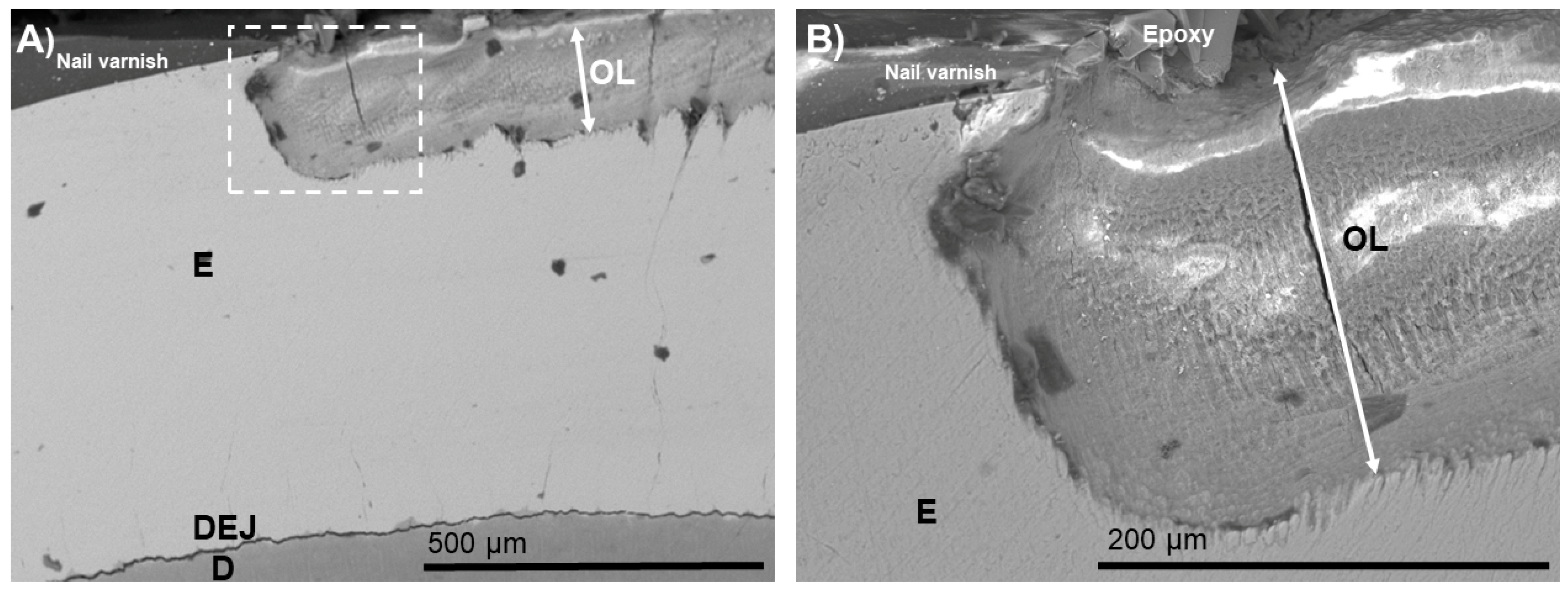This image contains two close-up microscope photographs of a sample, primarily showcasing regions labeled as "Nail Varnish" and "Epoxy". The left image, labeled "A", features a large, light gray area with a dotted square outlining a section highlighted with the word "Nail Varnish". Inside this outlined section, there's a vertical label "OL" along with several black dots. Additional labels within this image include "TEJ" above another "T" and "500 micrometers" on the far right. On the right side, image "B" provides an even closer view of the outlined area from image "A", indicating the same "Nail Varnish" but with enhanced focus on the features within, including the vertical "OL" and additional text "Epoxy" at the top, and "200 micrometers" at the bottom. The images reveal contrasting shades of dark and light gray with various annotated labels and measurements that highlight specific microscopic details of the sample.